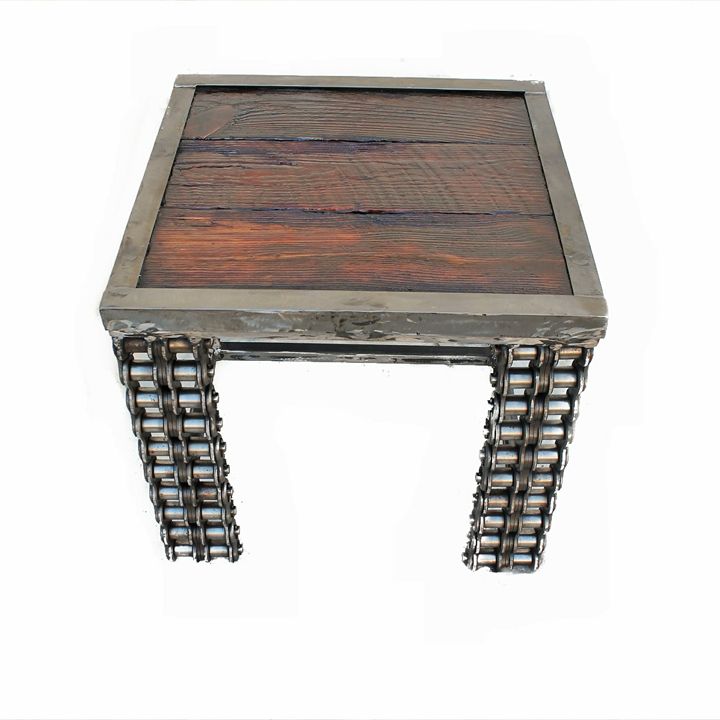The image showcases a small, narrow coffee table set against a solid white background, photographed at a top-down diagonal angle. The table features an intriguing and modern design with metal legs that resemble stacked rods or spools, somewhat akin to conveyor belts or tank tracks, giving them a jagged appearance. These silver legs support a tabletop composed of gray-colored wood, with three horizontal wooden slabs at its center. Each slab varies slightly in hue and texture, transitioning from a dark mahogany color to lighter, more washed-out tones. The table’s outer edge is framed in dark metal, enhancing its contemporary aesthetic. Overall, the table merges industrial elements with wood accents, creating a unique and striking piece of furniture.